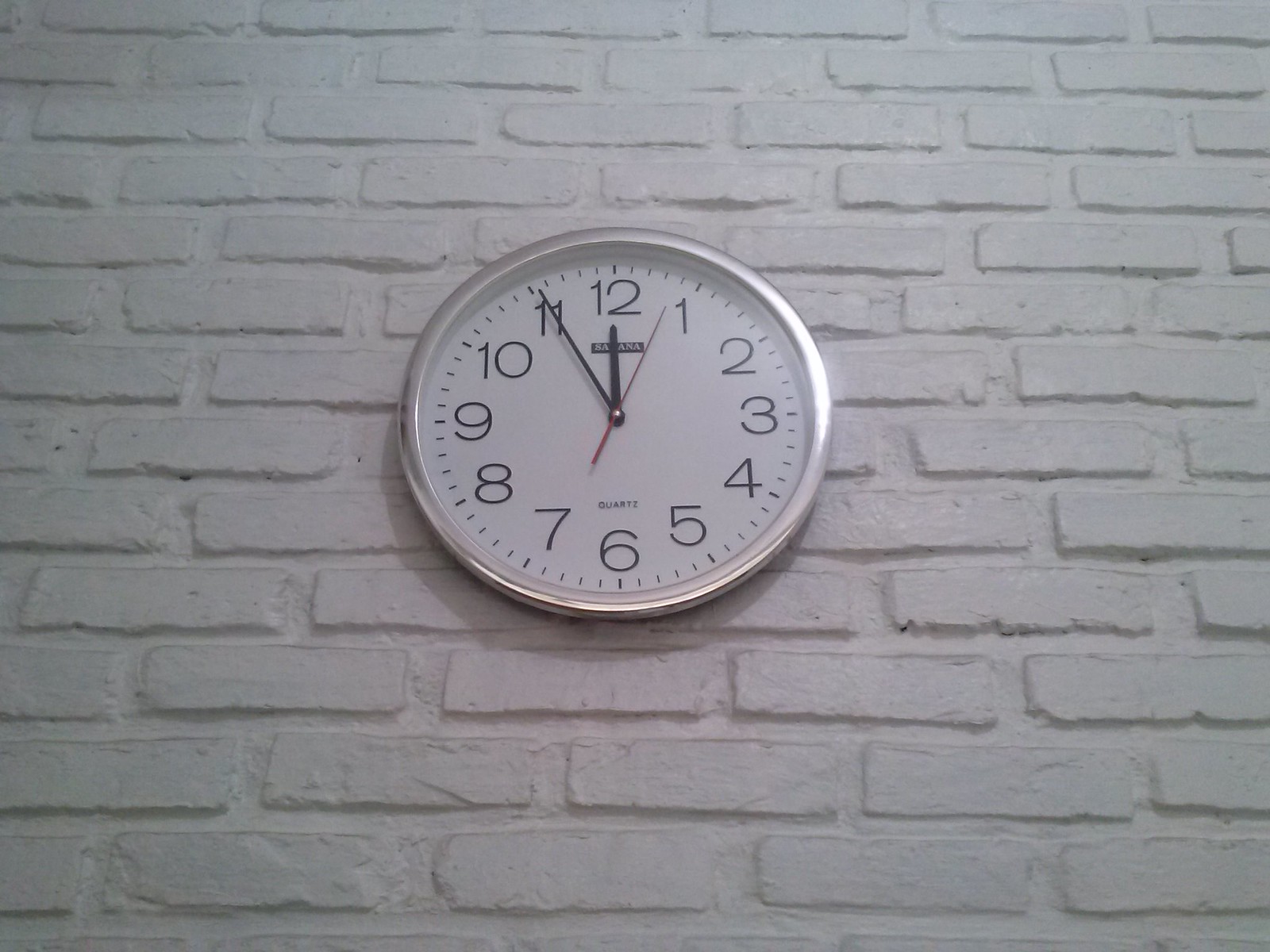This image captures a simple, traditional-style round wall clock mounted on an off-white painted brick wall. The bricks and the cement in between are uniformly coated in a single hue of off-white. The clock features a silver metallic border encasing a white face. Standard black numerals from 1 to 12 are arranged in a clockwise fashion, with "quartz" printed in black towards the bottom. The clock's hands include a black minute hand, a slightly thicker black hour hand, and an even thinner red second hand. The time displayed is precisely 11:55 and 4 seconds. The setting suggests a classroom or similar environment, although no other wall elements are visible from this vantage point.